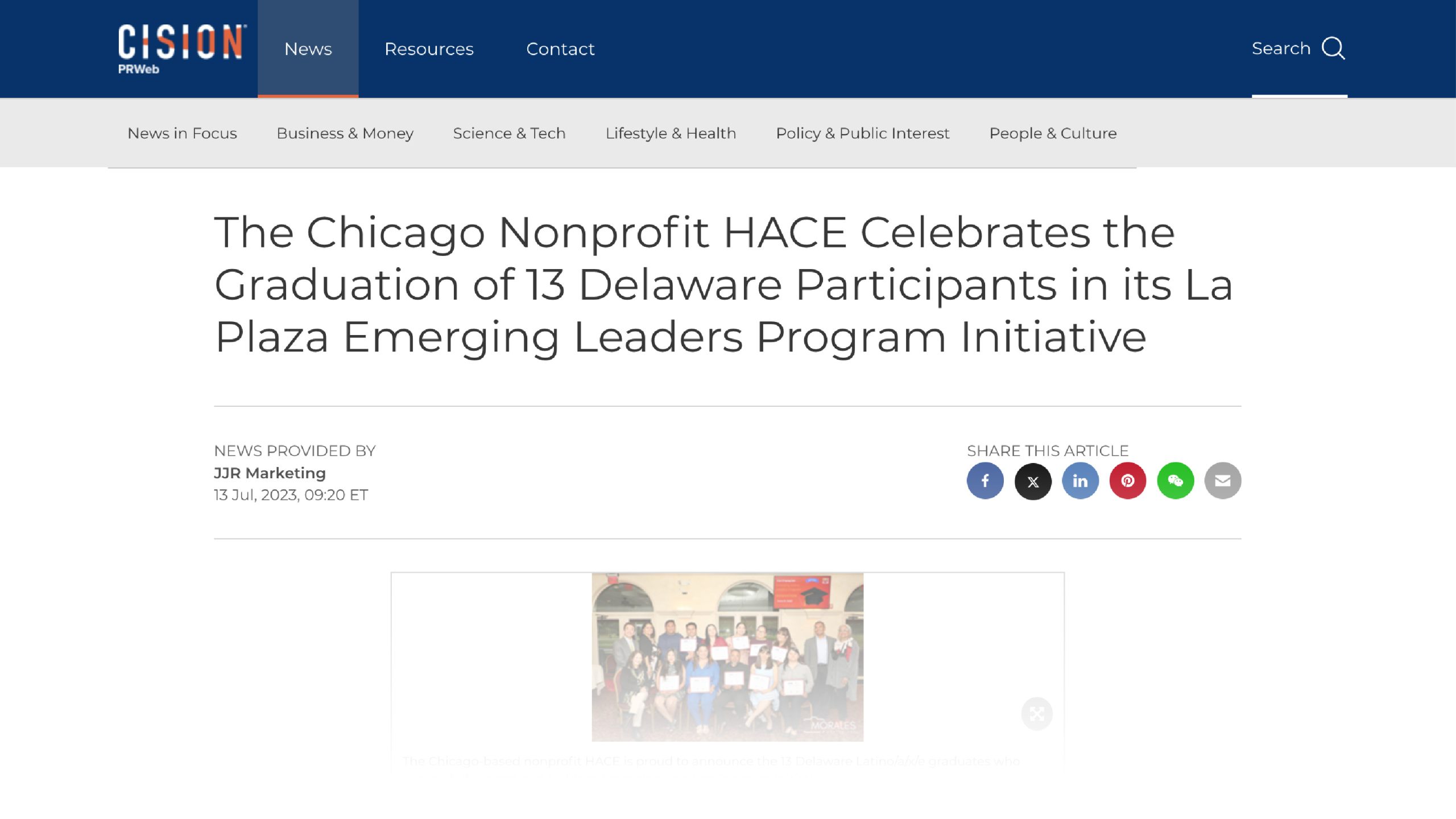The website in question is from Scission, prominently displaying the name "Scission" in white letters with an artistic red element that extends through the text, forming a triangular shape that doesn't quite meet the "C." Above the logo is a dark banner featuring navigation options: "News," "Resources," and "Contact," with a search bar situated on the right-hand side.

Beneath this is a gray navigation bar listing categories: "News and Focus," "Business and Money," "Science and Tech," "Lifestyles and Health," "Policy and Public Interest," and "People and Culture."

Further down, there is a headline about the Chicago nonprofit HACE celebrating the graduation of 13 Delaware participants from its LA Plaza Emerging Leaders Program initiative. Accompanying this is a partially obscured, whitewashed image of people congregating, likely the participants, but the details are faded and unclear.

Above the image is a long box labeled "News Provided By 33R Marketing," followed by the publication date. There are several icons and options for sharing the article on social media platforms, including Facebook and LinkedIn.